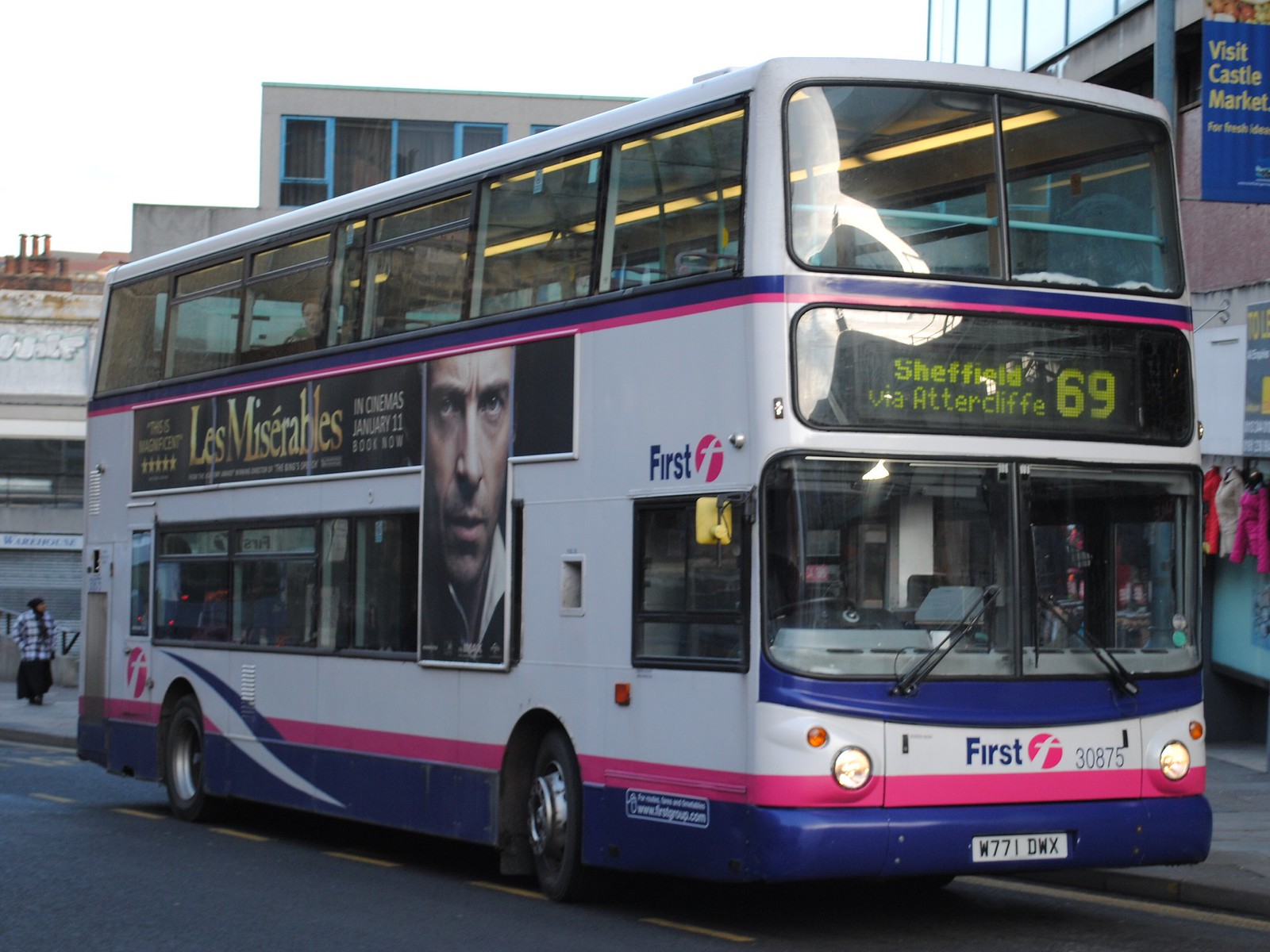This large square image prominently features a white double-decker bus with pink and blue stripes, positioned centrally on a city street. The bus, belonging to the "First" bus company, displays a circular pink F logo on both its front bumper and side. The digital destination sign at the front reads "Sheffield via Attercliffe" with the route number 69. The bus ID number, 30875, and license plate, W771DW6, are clearly visible. A banner on the side of the bus advertises "Les Miserables in cinemas, January 11th, Book Now," featuring an image of Hugh Jackman. Surrounding the bus, the backdrop includes various buildings with a distinct yellow sign stating "Castle Market" visible. The scene captures a portion of the sky, appearing white, in the top left corner. The road, composed of gray asphalt, runs beneath the bus. On the far left sidewalk, one person wearing a coat and a black skirt is visible. The photo seems to be taken during the day, giving an overall urban atmosphere.